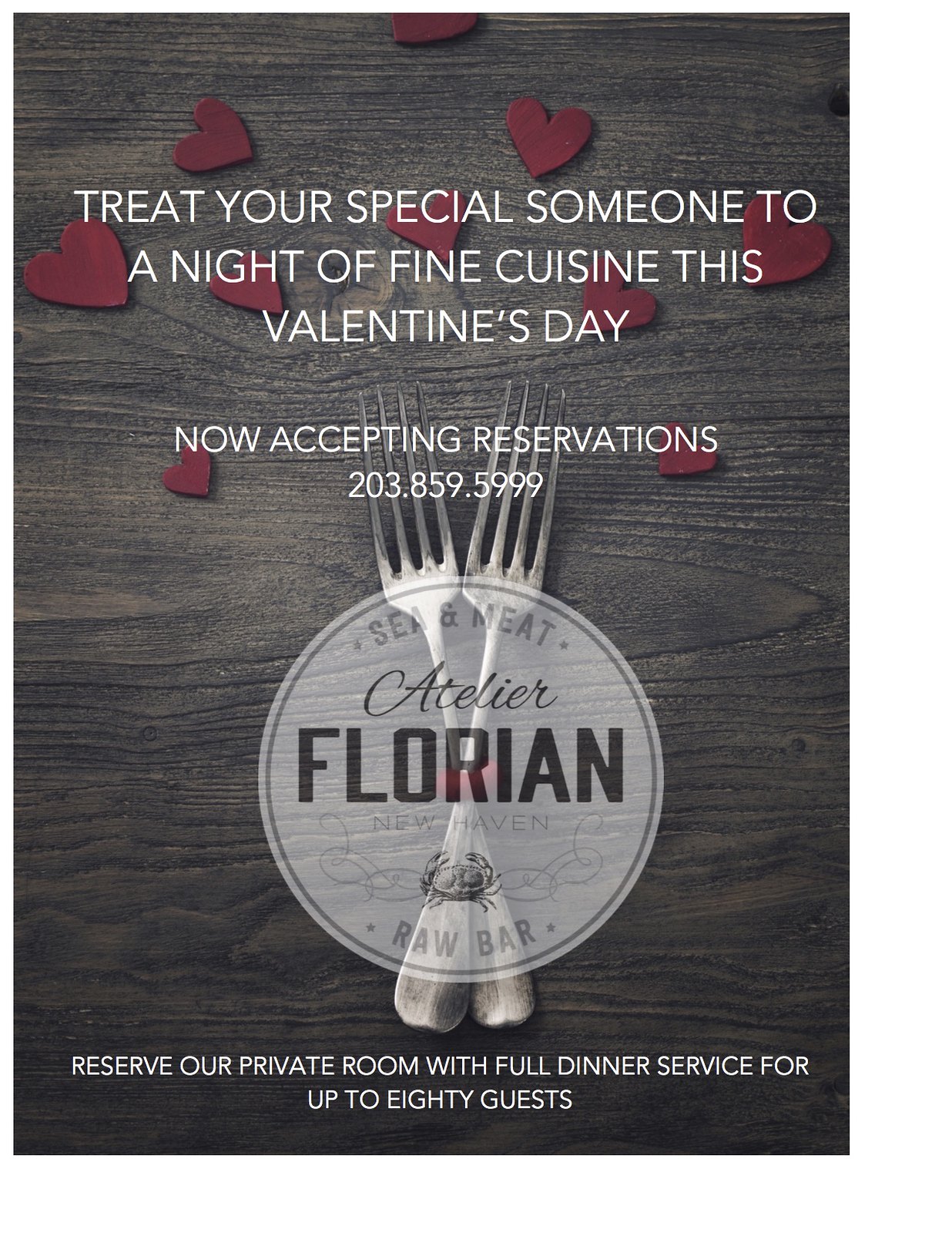This advertisement, likely from a website or magazine, features a dark-stained wooden table as the background, with distinguishable horizontal wood grains. At the very center, two forks are crossed to form an 'X,' their tines pointed upward. Overlaying the crossed forks is a semi-transparent, circular logo in grey, containing the text "See and Meet Atelier Florian Raw Bar" along with a small crab symbol. Scattered around the forks are small, three-dimensional red hearts casting subtle shadows. From top to bottom, centered in white text, the ad reads: "Treat your special someone to a night of fine cuisine this Valentine's Day. Now accepting reservations 203-859-5999. Reserve for our private room with full dinner service for up to 80 guests."